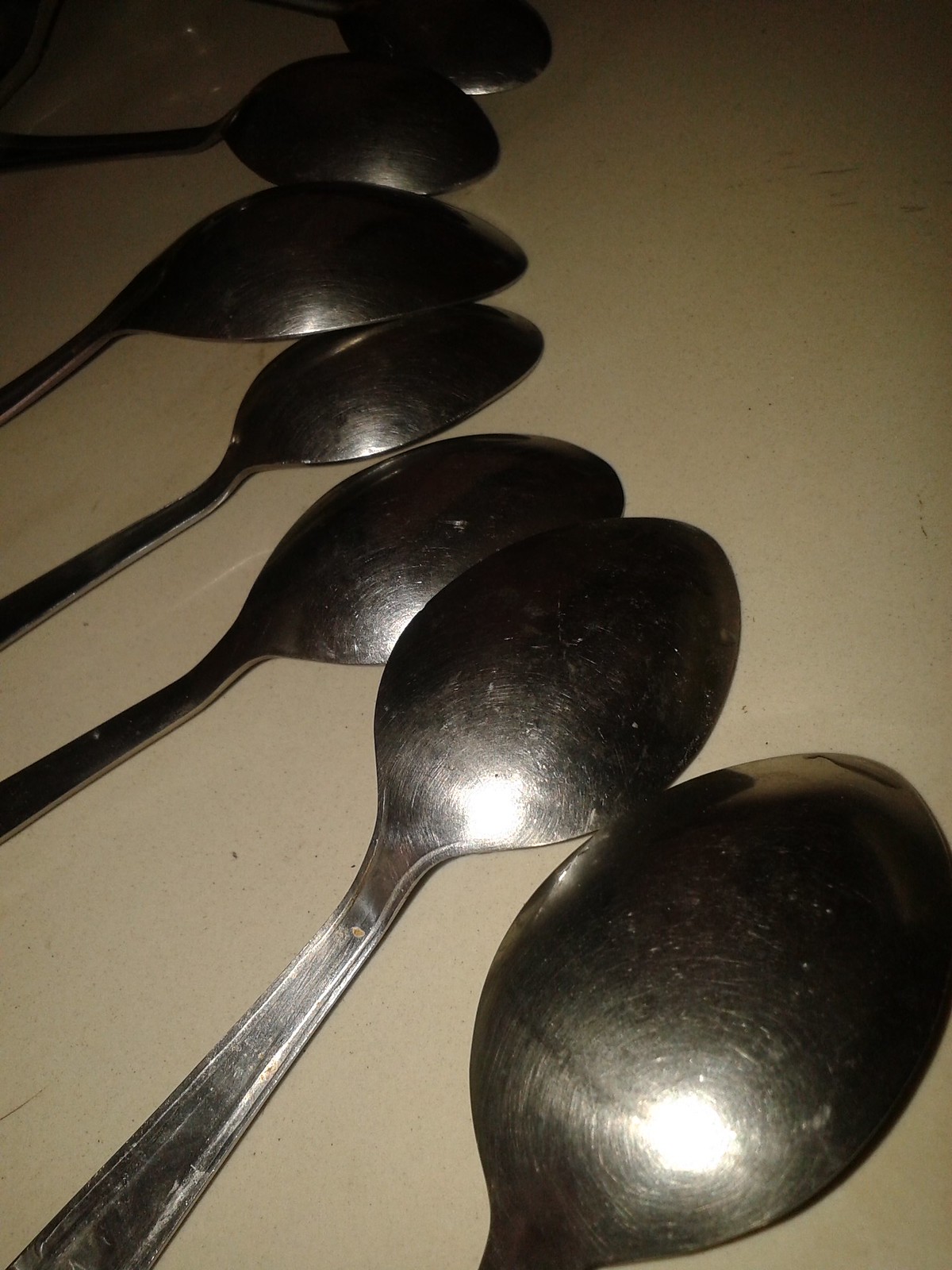This photograph captures a slightly-curved row of seven stainless steel spoons, laid face down on a smooth, white tabletop that appears grayish due to the lighting. Arranged in a slightly curved line that mimics a vertical smile, the spoons mostly rest adjacent to one another, with some slight overlapping. The handles of the spoons are cropped out by the edge of the image, so only the heads are visible. Most spoons feature reflections of overhead lighting, creating small spots of white glare. Although they are used and appear somewhat scuffed, with fine scratches visible on the closest spoons, they remain functionally clean. The second spoon from the bottom shows signs of additional dirt. The tabletop itself is speckled with small black dots, adding texture to the otherwise smooth surface, and there is slight vignetting in the upper corners of the image.